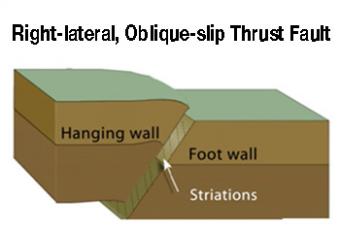This image is a detailed diagram on a white background, demonstrating a right lateral, oblique-slip thrust fault. The diagram is divided into several colorful, three-dimensional layers to illustrate the structure of the fault. 

At the top, a green layer represents the surface ground. Beneath it lies a golden-brown layer, labeled "Hanging Wall" on the left side, indicating the upper portion of the fault. The fault line is clearly visible, showing a distinct separation between the hanging wall and the "Footwall," which is labeled on the lower right side beneath the fault.

The bottom layer of the diagram is a dark brown stratum labeled "Striations," highlighting the directional movement along the fault. An arrow indicates the direction of the slip, with the upper section on the left side of the fault plane and the lower section on the right. The diagram effectively illustrates the complex nature of an oblique-slip fault in a visually engaging and educational manner.